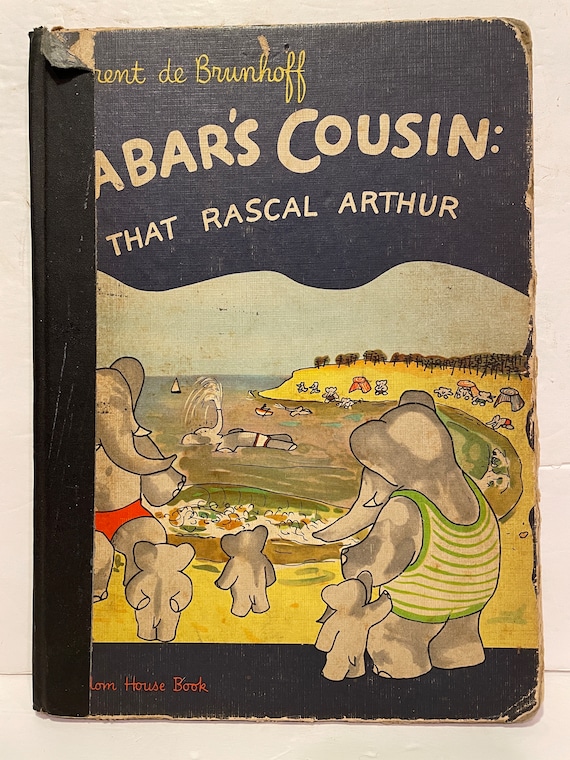The image depicts a well-worn, old children's book titled "Babar's Cousin, That Rascal Arthur." The hardcover book features visible signs of age and damage: its edges are worn, the corners are peeling, and there are small tears along the right side. The spine has been repaired with black tape, obscuring part of the title. The cover illustration portrays a vivid beach scene with Babar the Elephant, his cousin Arthur, and three little baby elephants enjoying the yellow sand. Arthur, wearing red swim trunks, and Babar, dressed in a green and yellow striped swimsuit, are prominently featured. One elephant is lying on its back in the water, playfully squirting water from its trunk, while small sailboats and canoes float in the background. Tents and chairs are scattered along the beach, and distant umbrellas complete the scene. The background appears as if the book is propped against a cement wall with outlines of painted bricks, giving a sense of a school setting. The cover's artwork is slightly torn on the left side, revealing the book's black underlying cover. At the bottom of the cover, partially obscured text reads, "house, book," against a black border.